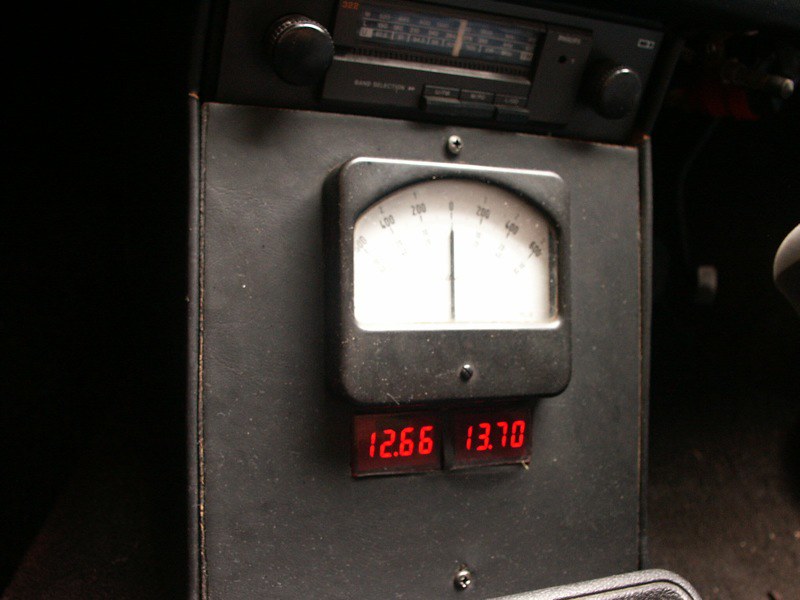This photograph captures a vintage piece of electronic equipment, characterized by its worn and scuffed appearance. At the top, there is a section of black plastic that features a classic radio tuning bar. Due to the blurriness of the image, the exact numbers on this bar are indistinguishable, but a light red bar is visible in the middle, reminiscent of the tuning indicators on old radios. Flanking this display are round, shiny black tuning dials. Additionally, there are three rectangular push buttons on this section, each with some unreadable white writing, further contributing to its old-fashioned look.

Below this, or possibly part of a separate device, is a rectangular black display case, likely made of heavily scuffed gray leather. The display mimics the style of vintage car dashboards and includes a needle that moves from left to right. The white face of the display has numbers marked from 400 on the left, to zero in the middle, and then ranging from 200, 400, to 600 on the right. The needle itself is either black or dark gray. Mounted above and below this face are two screws—one is a flathead, and the other a Phillips head.

At the bottom, there are two small rectangular digital displays with neon red numbers. The display on the left shows 12.66, while the one on the right reads 13.70. Another Phillips head screw is situated at the bottom of the object. Overall, the equipment presents a nostalgic aesthetic, indicative of its age and use.